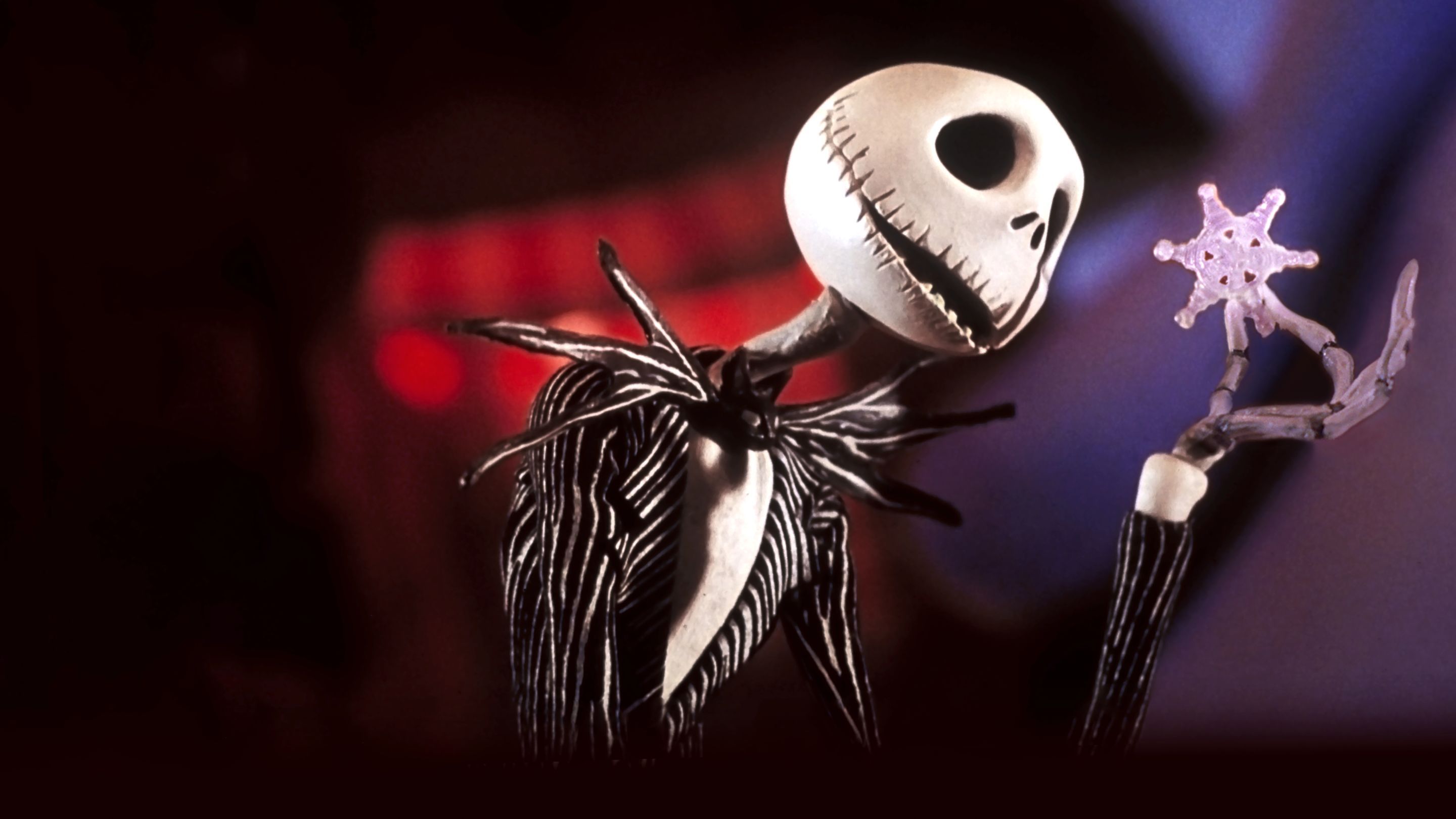The image depicts a detailed claymation of Jack Skellington, a character from "A Nightmare Before Christmas." Jack is standing at the center, predominantly visible from his upper body and head. He sports a distinctive black and white striped suit over a white shirt. His skeletal face, characterized by hollow eyes, a large mouth slightly ajar, and a hollow nose, is both sinister and intriguing. His left hand, resembling skeletal bones, is raised with his index finger and thumb delicately holding a small, clear snowflake with six points. The background is blurry, featuring an array of colors including dark purple, red, and black, adding to the eerie atmosphere without distracting from Jack’s detailed and charismatic form.